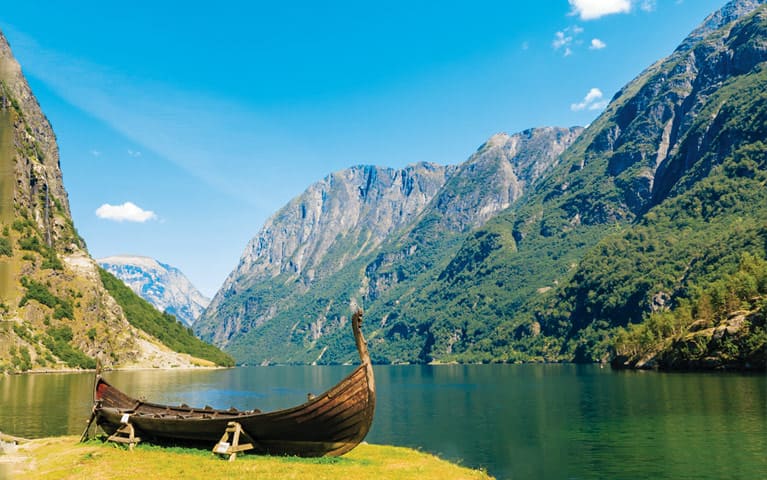This captivating photograph, taken in horizontal orientation, captures a serene river meandering through majestic mountains. The river exhibits a stunning greenish-blue hue, mirroring the verdant, tree-coated mountains that enclose it. The peaks of these mountains gradually transition into rocky terrain, but lower down, they are densely clothed in various types of green vegetation. 

Dominating the foreground of the image, slightly off-center to the left, is a handcrafted wooden vessel resembling an old-fashioned canoe or a Viking boat, distinguished by its prominent, curved prow that rises higher than modern canoes. This detailed decorative element—a stick-like structure—arches from the front, adding a historic charm to the scene. The boat rests on wooden stands, which stabilize and elevate it from the grassy ground, giving it a sense of careful preservation.

The sky above is a vivid, deep blue, punctuated with a few fluffy, white clouds, enhancing the brightness of this beautiful, sunny day. The collective elements of clear skies, rugged yet verdant mountains, tranquil reflective waters, and the nostalgic wooden boat come together to create an exquisitely detailed and picturesque landscape.